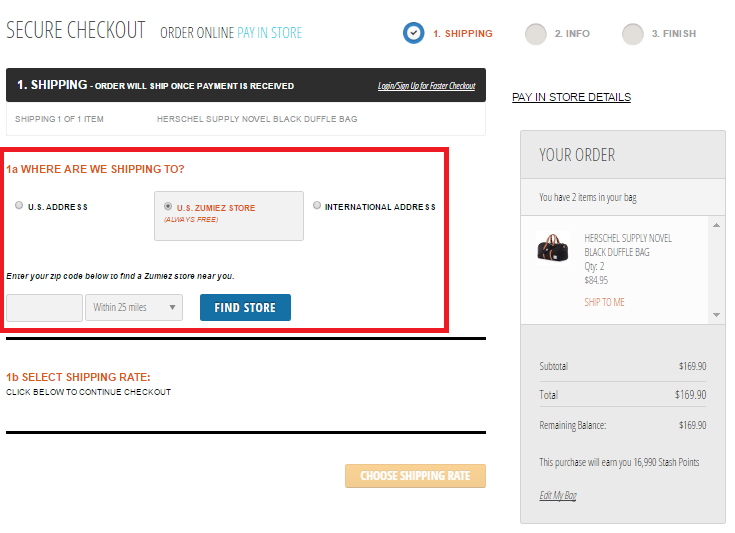The image presents an online checkout interface with various sections and instructions for completing a purchase.

At the top, the image features a white background with bolded text in uppercase letters that reads "SECURE CHECKOUT." Following this, also in uppercase, it says "ORDER ONLINE," and then in gray text, "PAY IN STORE."

On the right side, there's a blue circle containing a black checkmark, and next to it, in black text, it states "FREE SHIPPING." Below this are two gray circles, one labeled "2 INFO" and the other "3 FINISH."

Next, a black background section contains white text that reads "1 SHIPPING: Order will be shipped once payment is received." Underlined beneath this, it says "Log in / Sign up for faster checkout."

Continuing on a white background, gray text indicates "SHIPPING 1 OF 1 ITEM: HERSCHEL SUPPLY NOVEL BLACK DUFFEL BAG." A red rectangle appears below this section with a white center, and inside in red text, it reads "1A WHERE ARE WE SHIPPING TO?" The options provided are "USA, US ADDRESS, or US ZÜM STORE" highlighted in a grayish color, or "INTERNATIONAL STORE."

Beneath these options, in blue text, it instructs, "Enter your ZIP code below to find a Zum store near you," accompanied by a gray input field to enter a zip code, set within a 25-mile radius. Next to this input field is a blue button with the white, bold text "FIND A STORE."

Following this, under the title "1B SELECT SHIPPING RATE," text in brown or black instructs to "Click below to continue checkout." On the right-hand side, there's an additional mention of "PAY IN STORE."

Lastly, the price of the black bag is displayed in gray text, listed at $169, with the note that this is considered to be "a complete and utter ripoff."